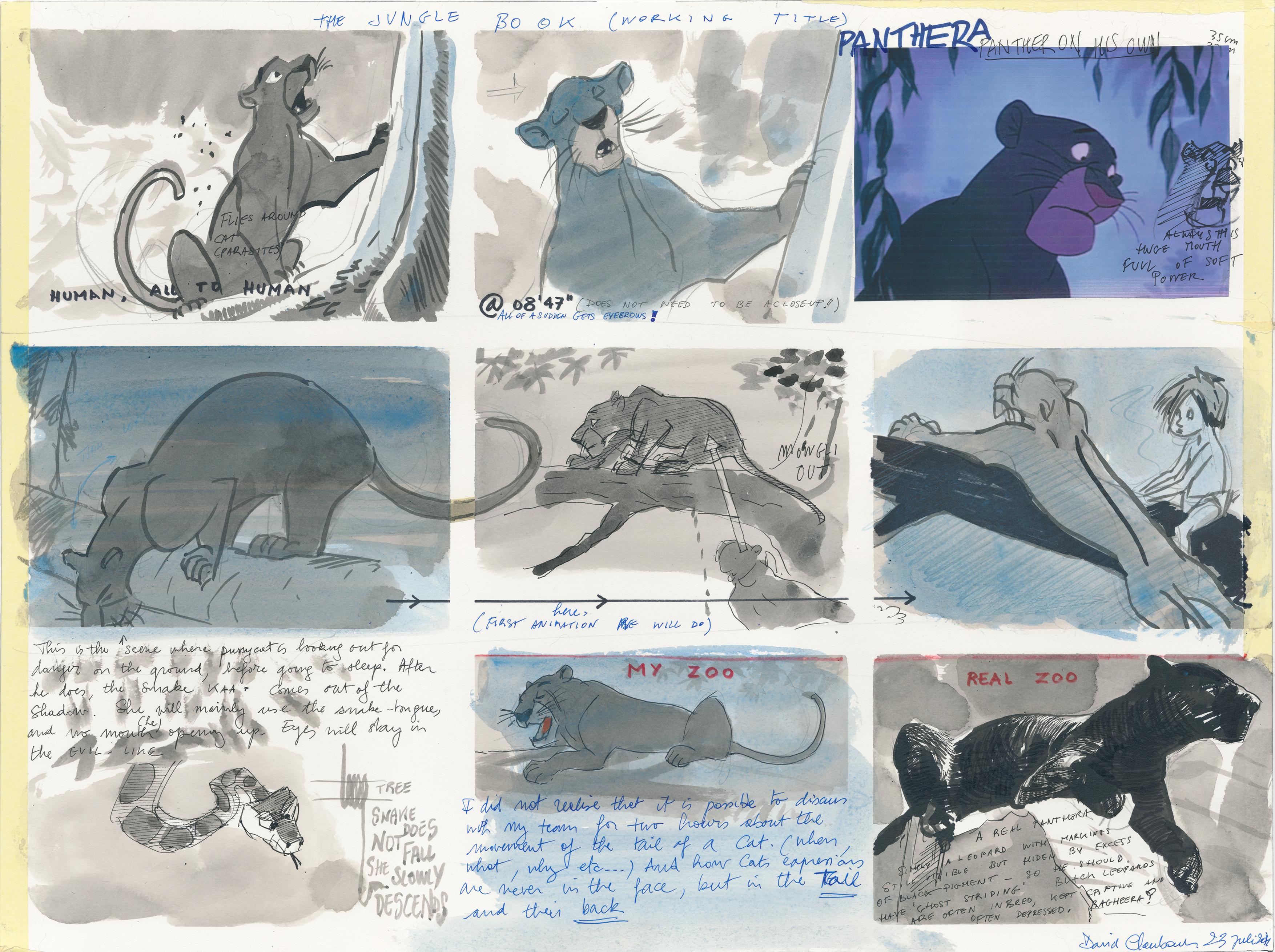This image illustrates an early draft of a cartoon strip, tentatively titled "The Jungle Book" as noted in scratchy handwriting at the top of the white page. The primary character depicted across the image is a panther, referred to as Panthera, rendered in pen and ink. The sketch framework consists of three rows, each containing three panels that showcase various scenes involving the panther character in hues of gray, blue-gray, and darker shades suggesting nighttime settings. Notably present in the middle panels are minimal yet poignant scenes: one featuring a little boy and the panther against a log and tree, and other bottom panels inscribed with "My Zoo" and "Real Zoo" in red ink. Completing the scene is a detailed portrayal of the panther lounging across a notebook filled with handwritten text. Although the exact handwritten text is largely illegible, these notations likely describe the scenes in the panels. Clearly a work in progress, the sketch exudes an essence reminiscent of classic Disney character illustrations and meticulously captures the foundational elements of the iconic Jungle Book narrative.